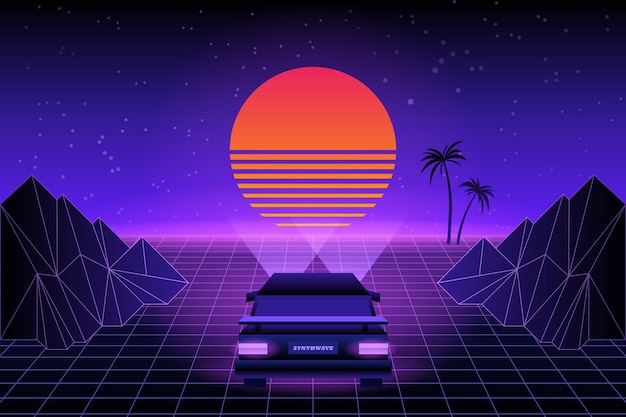In this detailed, computer-generated digital artwork, a sleek black sports car with a raised spoiler dominates the foreground. The car's license plate reads "Synthwave," and its taillights and headlights glow a light purple hue, casting an otherworldly light. The vehicle sits on a black grid-patterned surface, partitioned by thin gray stripes into rectangular sections, creating a sense of depth and digital precision.

The sky above transitions from evening to twilight, awash in deep blue hues punctuated by tiny gray circles representing stars. A large luminescent sun looms prominently, its top half solid orange while the bottom half is composed of horizontal orange stripes, revealing the blue sky through varying lengths. Flanking the sun on either side are digitally rendered, dark gray mountains with light gray outlines, featuring distinct triangular shapes. Additionally, two palm trees ascend on the right side, adding a touch of organic contrast to the geometric landscape. This intersection of vibrant colors and sharp lines evokes a retro-futuristic, 'inside a computer' ambiance, encapsulating the essence of Synthwave aesthetics.